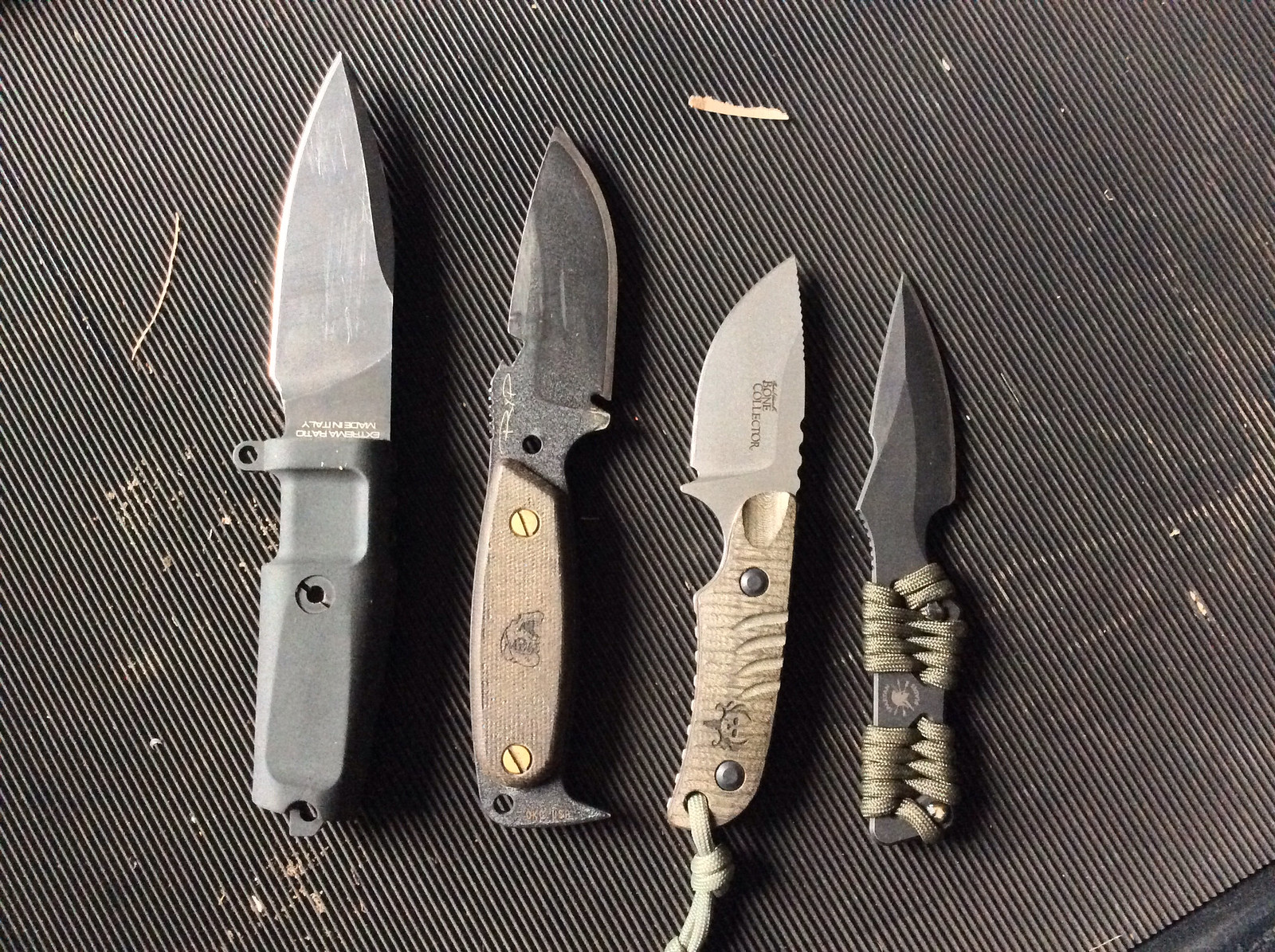The photograph shows four utility knives arranged side by side on a black, ridged rubber mat that is scuffed and dotted with dirt and debris. The mat's black surface has close-set striations running diagonally from the top left to the bottom right, with lighter beige areas where dirt has accumulated and the surface has been worn down. From left to right, the knives vary in size and design. 

The first knife is the longest, with a short, pointy blade and a gray handle. The handle shows a partial inscription that reads “Extremes” and “Made in Italy.” The second knife, which faces the right, has a slightly flatter blade with a light wooden handle secured by two visible bronze screws. The knife also features a tool etched into the blade and a ripping tool at the bottom. The third knife, shorter than the first two, has a silver blade marked with "Bone Collector" and a beige handle adorned with a skull motif. This one also faces left. The fourth and smallest knife has a black blade and a metal handle wrapped in green paracord, giving it a military look. All four knives appear robust and practical, ideal for outdoor or wilderness use.